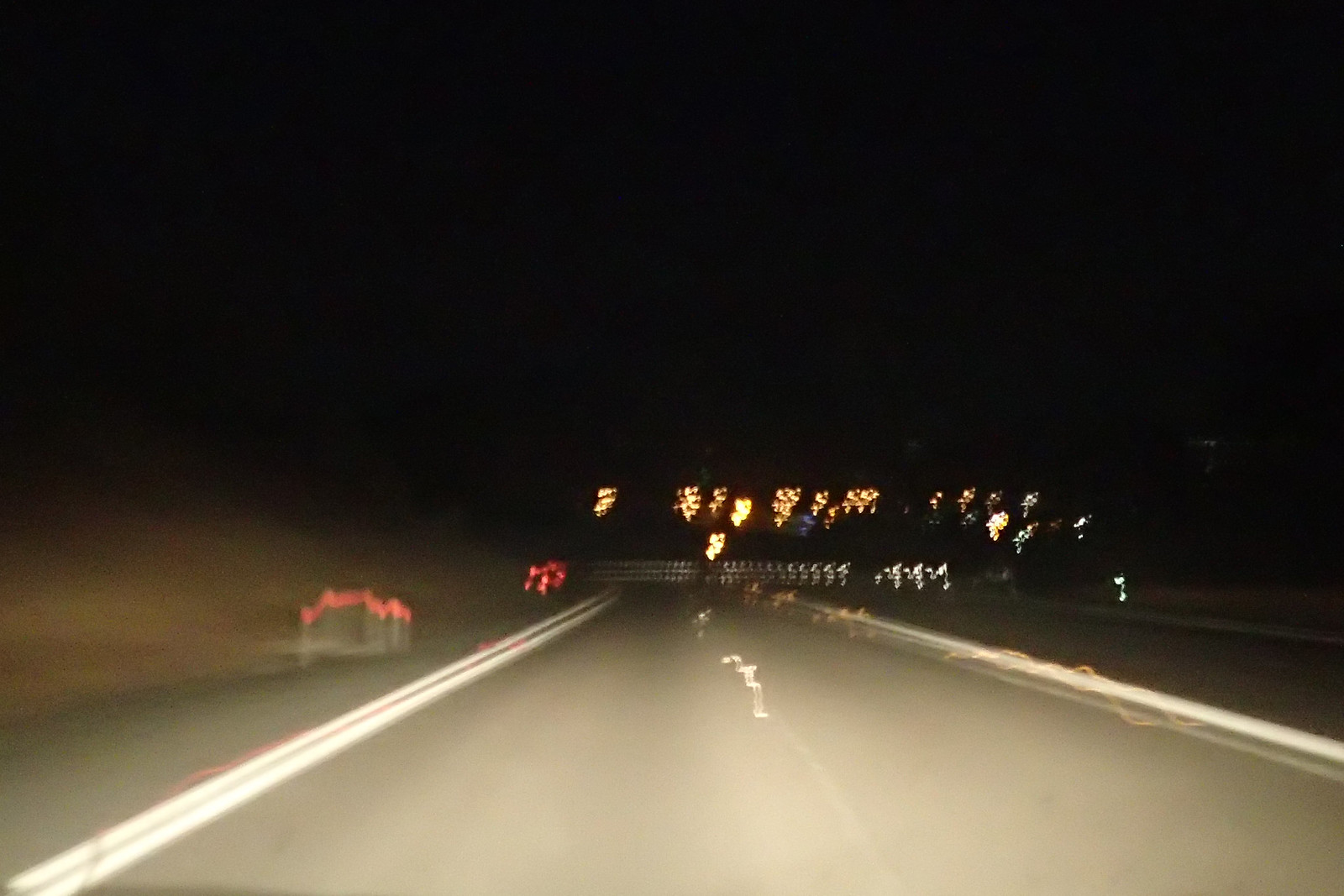A blurred nighttime photograph taken from either inside a car or by a person standing on a road or highway. The viewer's perspective is straight down the road, with distant streetlights casting faint glows. There is a guardrail on the right side of the image, reflecting some of the streetlight's illumination. The road markings include double white lines on the left and a single white line with a yellowish smudge along the right. On the left side, there are small warning signs or perhaps a railing. The sky occupies the top two-thirds of the image and is a deep, uninterrupted black, adding to the night setting's obscurity.